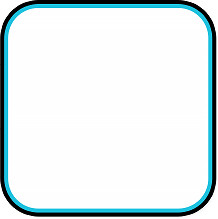The image is a small digital drawing depicting a minimalist design. It features a symmetrical, white-filled square with highly curved, beveled corners, approximately one to one and a half inches in size. Surrounding the white interior, there's an inner border of bright light blue, and around this blue border, a thin, slightly jagged black outline. Both the light blue and black borders are of equal, fine thickness. The overall depiction is a clean, three-color palette comprising white, light blue, and black, with a consistent symmetry in the curved corners. The white interior might show faint lines or a ghost image upon closer inspection, suggesting the background of a digital document.